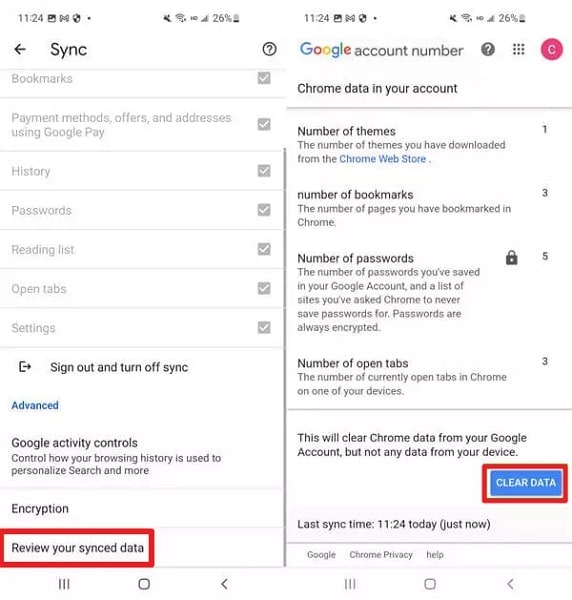The image displays two settings screens on an Android phone, arranged side by side. 

**Left Screen:**
- **Time and Status Bar:** The time reads 11:24. Icons at the top include a picture icon, Google Mail icon, a security icon, battery percentage at 26%, and a good network signal with four out of five bars and an HD indicator. The sound is muted.
- **Sync Settings:** The main content shows the sync settings. A sync icon (two arrows forming a circle) and a question mark are displayed at the top. Various settings are listed below, all in light gray with checkboxes marked, indicating they are active but not currently modifiable. At the bottom in black font, there are options to "Sign out and turn off sync" and an advanced settings link. Google Activity Controls, encryption, and reviewing sync data are highlighted in a red square.

**Right Screen:**
- **Google Account Details:** The screen shows details related to a Google account, labeled "C" in a red circle, with a question mark and ellipses for additional options.
- **Account Information:** This section lists several headings with corresponding data:
  - **Themes:** No specific number or detail provided.
  - **Bookmarks:** Three bookmarks.
  - **Passwords:** Protected with five passwords indicated by a padlock symbol.
  - **Open Tabs:** Three open tabs.
- **Data Management:** A note indicates that clearing data will remove Chrome data from the Google account but not from the device itself. A blue "Clear data" button is prominently highlighted in a red square.